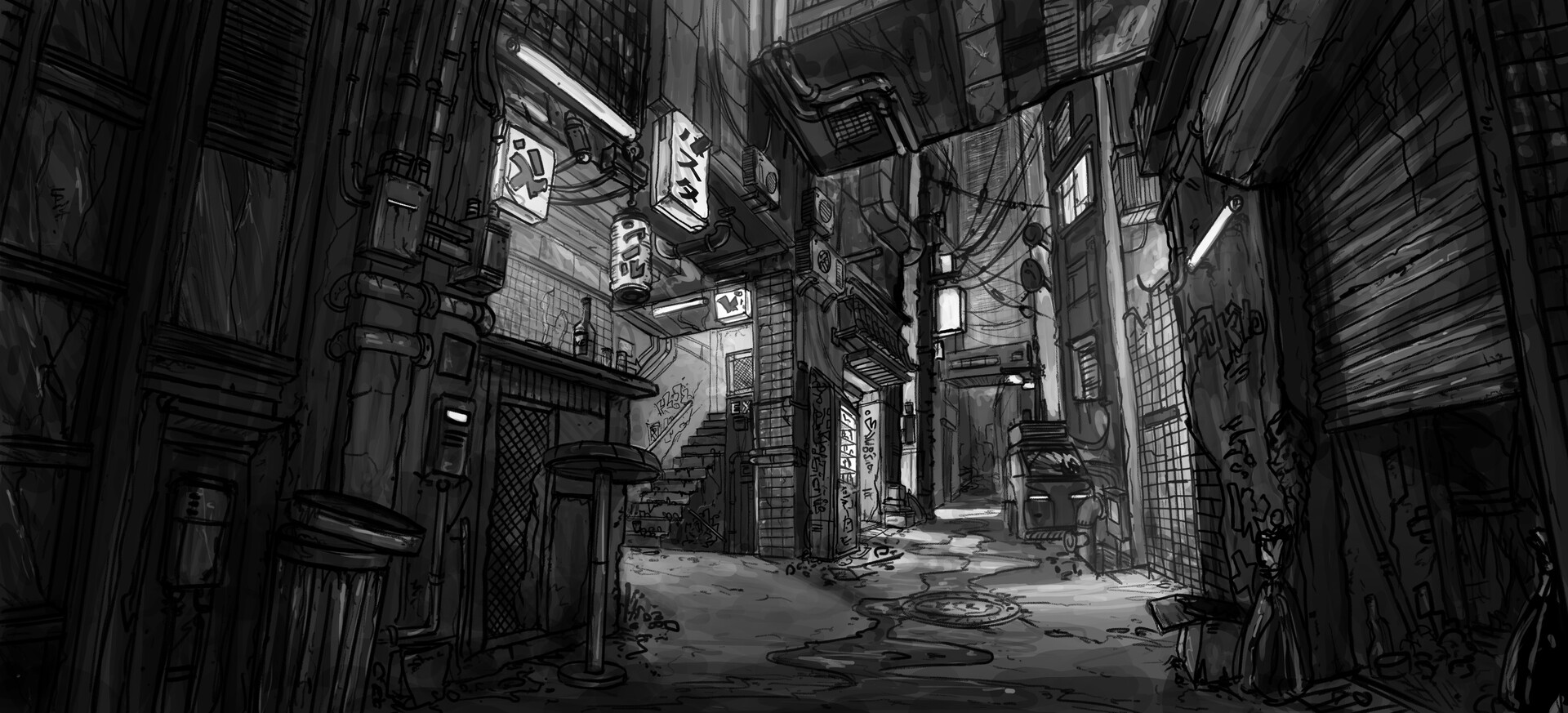This detailed black and white illustration depicts a desolate, futuristic alleyway in a city evocative of an anime or comic book setting. The scene exudes an ominous, shadowy atmosphere, with dilapidated buildings flanking either side of the narrow passage. In the foreground on the left, a trash can with its lid ajar sits next to a building adorned with piping and electrical boxes. Adjoining this building is a small shack, adding to the cluttered feel. A bar stool with a counter, housing a bottle of alcohol and a couple of glasses, suggests the presence of a neglected speakeasy or dive bar. Above this area, a cluster of illuminated signs bearing Asian characters—likely Japanese—hang from the ceiling and walls, hinting at the alleyway's possible location or influence.

On the right side of the alley, several buildings stand with boarded-up windows and a fence blocking off a side alley. Further down, a parked van is positioned across from an electrical pole and what appears to be a vending machine tucked into an alcove. The alleyway is littered with rubble, cracked concrete, and occasional puddles of stagnant water, emphasizing its neglected state. Towards the back, a staircase in a recessed alcove leads up to a door, which is potentially the back entrance to a restaurant or club, reinforced by the concentration of neon signs in the vicinity. Power lines crisscross above, and several windows on the second floor along the right side emit a dim light, contributing to the eerie, desolate ambiance of the setting. The artwork, likely created digitally, captures an enigmatic and sombre scene devoid of any human presence.